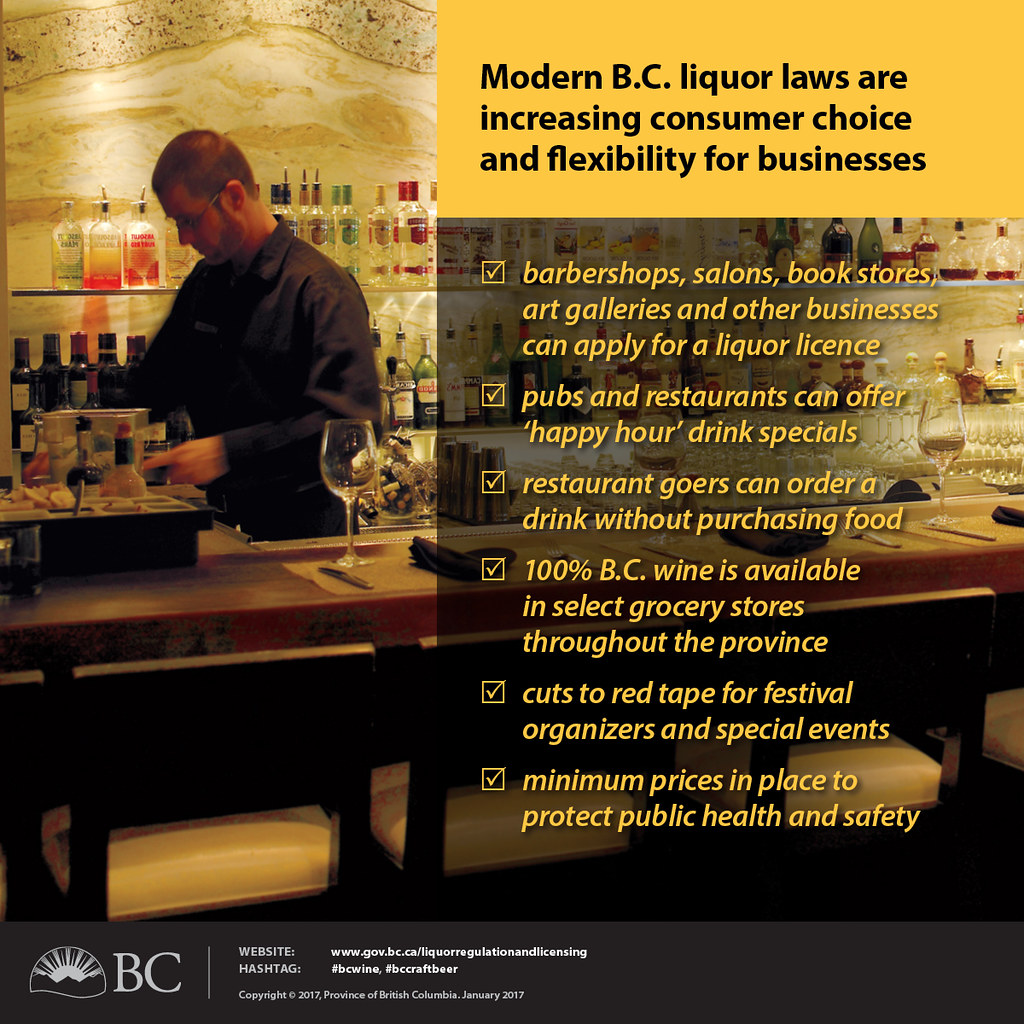The image depicts a promotional flyer created by the beer and wine craft brewers of British Columbia, with a predominantly yellow tone and a layout clearly divided into two sections. On the left side, a man with short brown hair and glasses, wearing a dark, long-sleeved black or grey shirt and black pants, stands behind a bar with a marbled-effect wall. He is intensely focused on preparing a cocktail, surrounded by a wine glass on the bar and an assortment of glassware and liquor bottles neatly arranged on shelves in the background. Beside him on the right side, there is a solid yellow-orange rectangle containing black text, stating "Modern BC liquor laws are increasing consumer choice and flexibility for businesses." Below this, a checklist with several specific points highlights the benefits of these new regulations, including the ability for barbershops, salons, bookstores, and art galleries to apply for liquor licenses; happy hour specials in pubs and restaurants; the option for diners to order drinks without needing to purchase food; the availability of BC wine in select grocery stores; and streamlined processes for festival organizers. The lower part of the flyer has a dark grey border, featuring the BC logo with a sun graphic, the website address, a hashtag, and the copyright information marked as January 2017. The entire scene is set within a vibrant bar adorned with white and black stools.